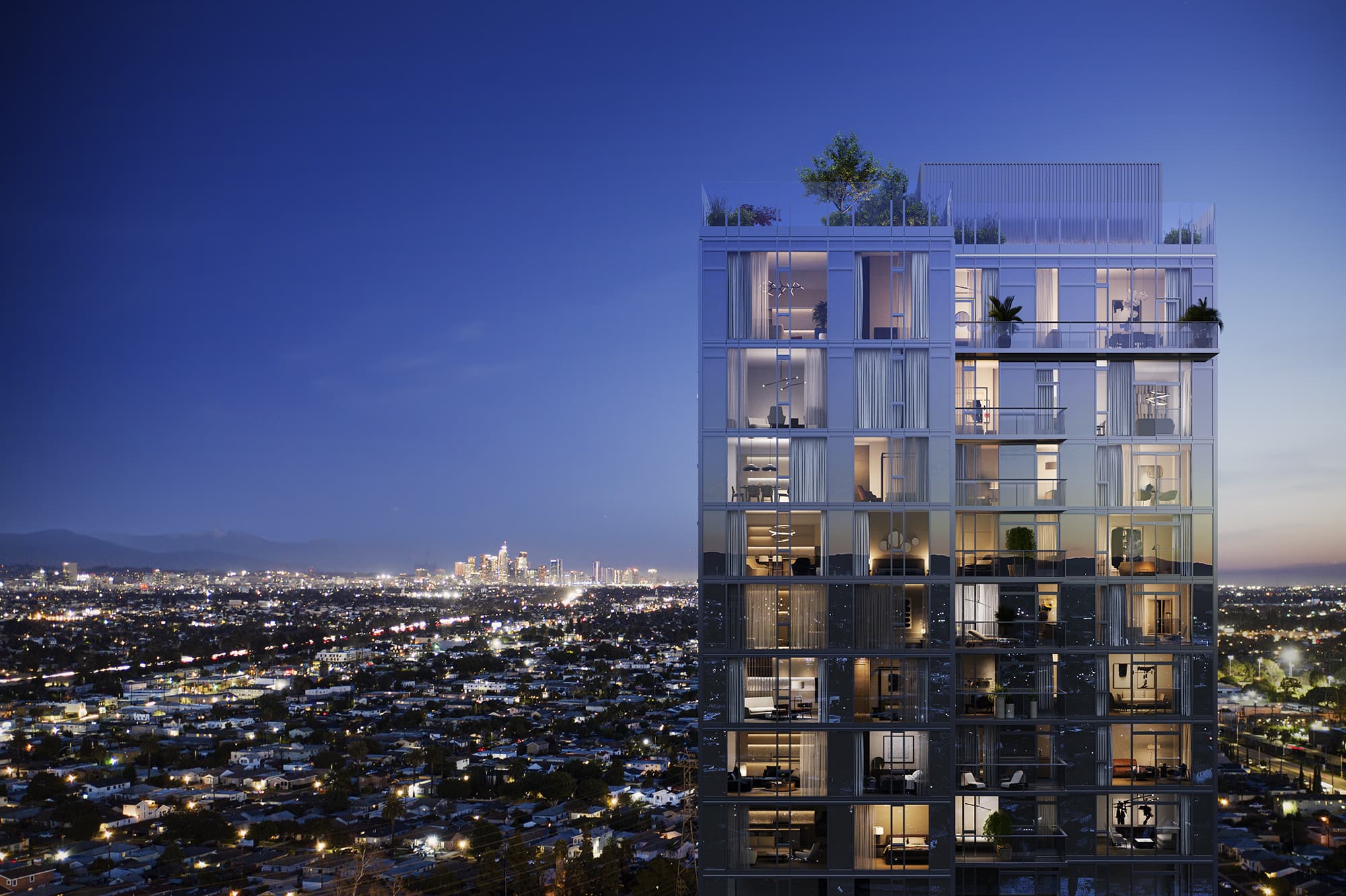This horizontal rectangular image, taken as an aerial view at night, captures a strikingly tall apartment building that stands prominently against the dark blue, nearly purple sky, amidst a backdrop of smaller buildings. The photograph, possibly taken from a drone or a nearby structure, showcases the cityscape with street lights illuminating main roads that stretch out into the periphery. The skyline in the distance reveals clusters of tall buildings, while in the forefront, the solitary towering apartment building dominates the scene. 

Each apartment features floor-to-ceiling glass walls and small balconies with vibrant plants, allowing a glimpse into the lit interiors. The rooftop is adorned with trees and encircled by a fence, adding a touch of greenery to the urban environment. The lights are almost entirely on, creating a luminous spectacle that contrasts with the night, emphasizing both the close-knit community within the building and the expansive, brightly lit city that surrounds it.